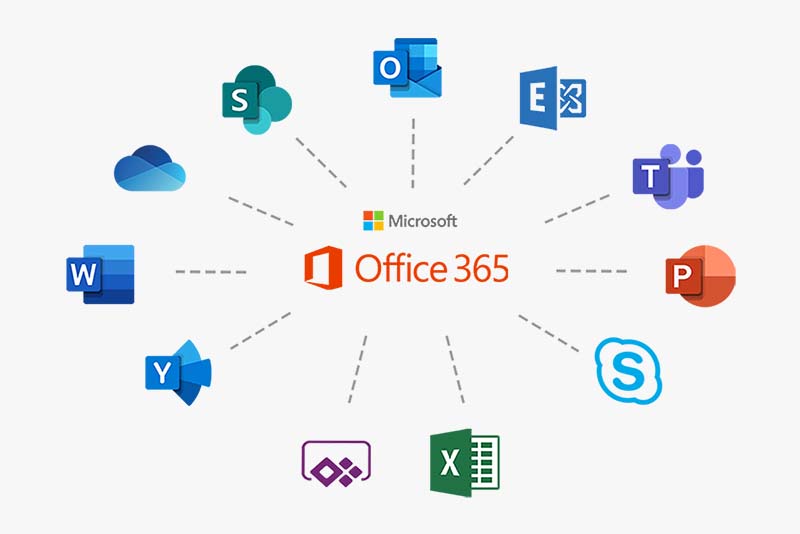The image depicts the Microsoft Office 365 suite, featuring icons of various Office applications arranged in a circular pattern surrounding the text "Office 365." To the left of the text, an orange square with an open side pointing left is prominently displayed. Above "Office 365" in smaller font is the word "Microsoft," accompanied by the Microsoft logo, which comprises four small squares forming a larger square.

The circle of application icons includes vividly recognizable symbols for Excel, Skype, PowerPoint, Word, and others, each connected by lines extending from the central "Office 365" text. Among the icons, there is an "O" indicating Outlook, a "Y," a "T," and a cloud icon, representing various facets of the Office 365 ecosystem. The overall layout skillfully highlights the comprehensive suite of tools available within Microsoft Office 365, symbolizing their interconnected functionality.